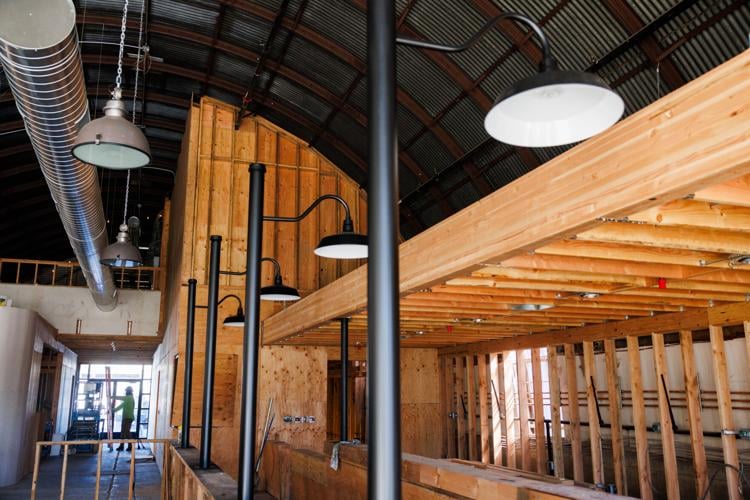The image depicts an expansive, partially constructed hall with a towering, semicircular roof that is predominantly dark, tinged slightly reddish at the beams. The room is filled with numerous wooden structures, including beams and slats, especially concentrated towards the back and top of the image, stretching horizontally from right to left and vertically towards the ceiling. Several black poles with overhead lights, organized in a single row, extend from the middle of the picture towards the background. Additional circular, white lights hang from the ceiling on the left side, accompanied by a silver vent pipe running along the ceiling's left side to the back. The right side of the space showcases dense wooden paneling and framing, whereas the left side is more open, revealing a distant construction worker managing a ladder or similar equipment. The room’s overall unfinished appearance, with visible building materials and structures, suggests it may become a commercial area such as a shop or lounge. Large silver pipes span the ceiling, reinforcing the construction site's incomplete state, while the far end reveals large glass doors with people standing nearby, implying active progress and development.